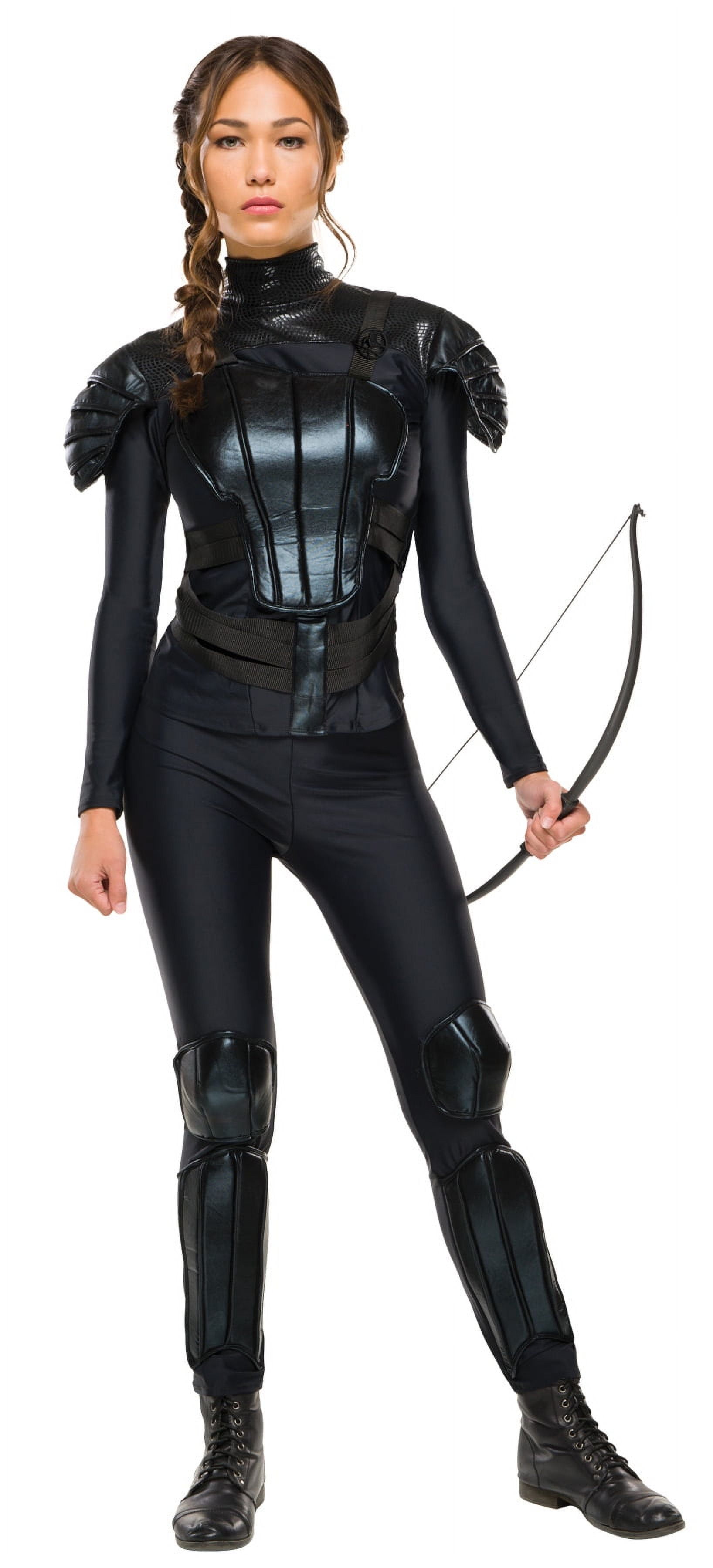In the image, a woman who remarkably resembles Jennifer Lawrence as Katniss Everdeen from The Hunger Games stands poised against a white background. She has brown hair, partially braided on one side, framing her face with small eyes, brown eyebrows, and pink lips. Her expression is serious, staring directly at the camera. She wears a predominantly black outfit, consisting of tight black yoga pants adorned with black kneepads and shin guards, black boots, and a top layered with shiny black armor, complete with shoulder pads and pleats on the chest area. In her left hand, she holds a black, curved bow with a thin string, ready for action. Her right hand is clenched in a fist, and her left leg is stretched out to the side, giving her a warrior-like stance.